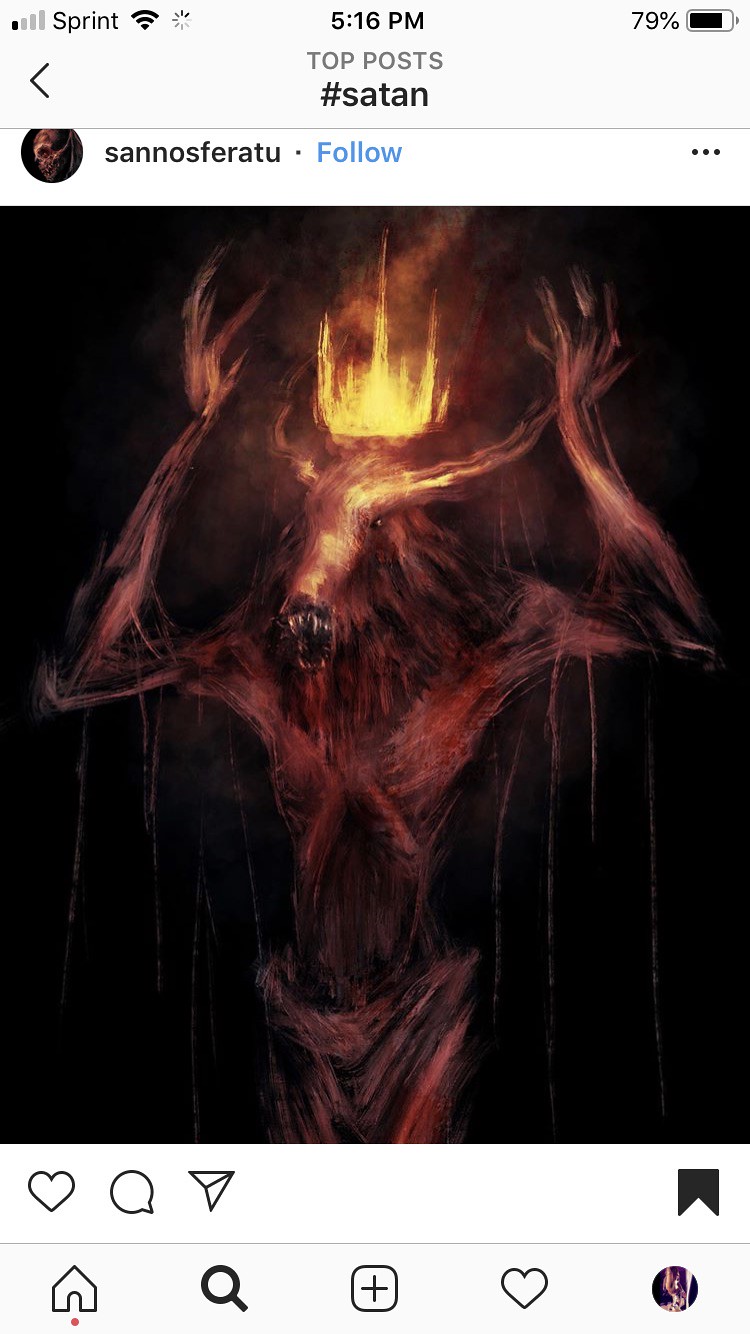This image is a digital rendering by the Instagram artist Sanosferatu, depicting a fantasy creature reminiscent of Satan under the hashtag #Satan. The creature, a dark and ominous figure, combines elements of various beasts such as a minotaur, horse, deer, and bear. It has a skeletal and wispy body marked with bloodstains and features a bull-like head with horns projecting above its eyes. The creature's mouth is open wide as if hollering, and atop its head, a crown of flames adds a sinister touch. The image, undoubtedly a piece of digital artwork possibly blended with oil-based techniques, was captured in an iPhone screenshot showing typical Instagram interface elements including the like, comment, share, and save buttons, along with account and post details.